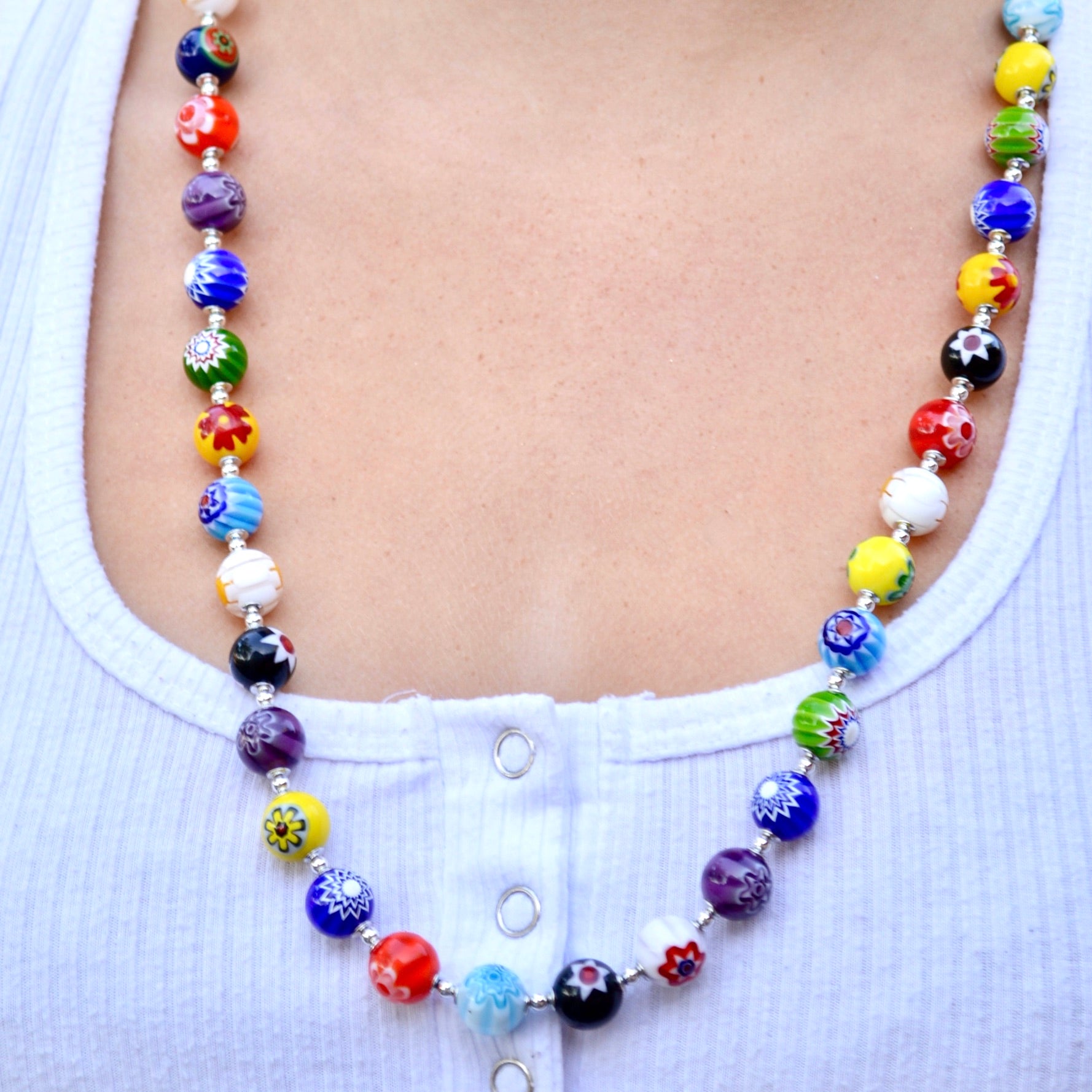This photograph focuses on a brightly colored, multi-beaded necklace draped around a woman's neck and chest, extending down to her sternum. The background features a white knit button-up shirt, exposing much of her mid-chest and clavicle area. The shirt has three visible silver snaps running down the center. The necklace consists of a variety of beads in colors such as blue, red, yellow, green, purple, and white, each separated by small metal beads. The beads themselves are intricately designed, showcasing flower and sunburst patterns that resemble marbles.